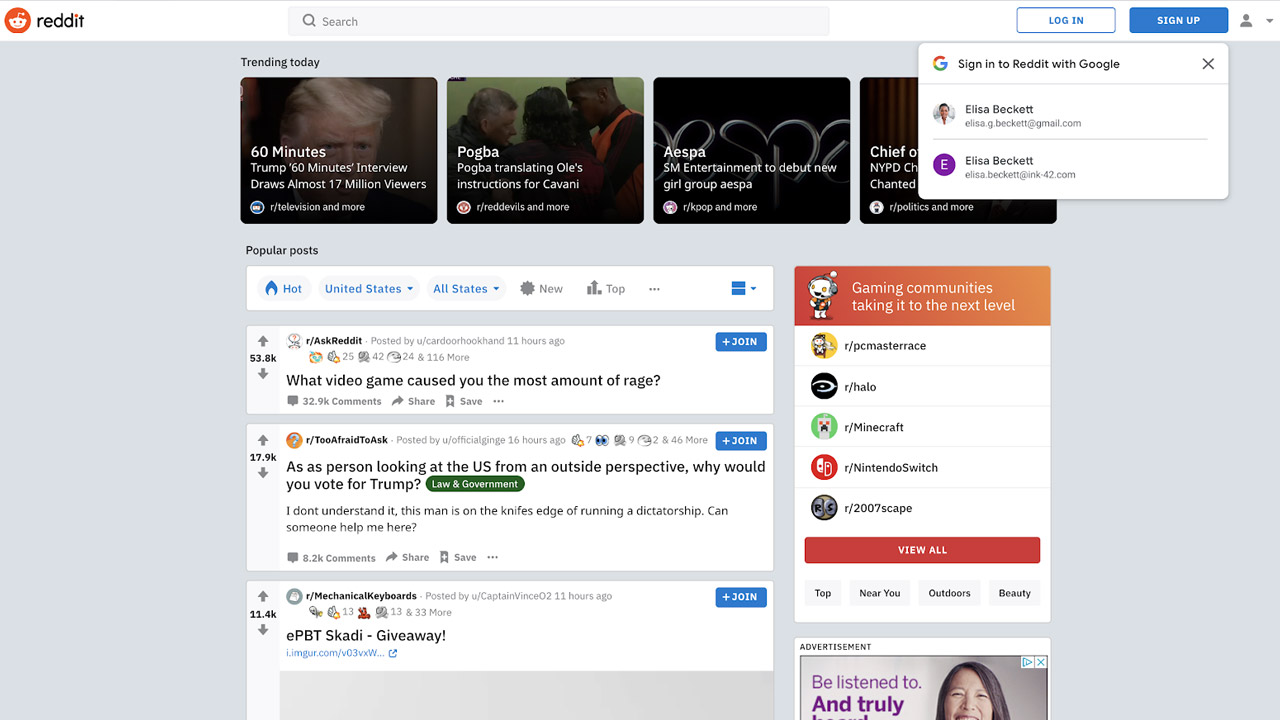**Detailed Caption for Reddit Homepage Screenshot**

The image is a screenshot showcasing the Reddit homepage. In the top right corner of the screen, the "Login" and "Sign Up" buttons are clearly visible, suggesting the user has not logged into their account. Along the upper portion of the page, there is a "Trending Today" section featuring four box icons, each with an accompanying image and title providing a snapshot of trending topics. The listed trends include "60 Minutes," "Pogba," "AES Spa," and a partially visible "Cheap Something."

Dominating the central area of the homepage are the current popular posts, with the top three headlines prominently displayed. The first post is titled "What Video Game Caused You the Most Amount of Rage?" The second asks, "As a person looking at the U.S. from an outside perspective, why would you vote for Trump?" The third headline reads "EPBT Scatty Giveaway."

On the right side of the page, a highlighted section labeled "Gaming Communities Taking It to the Next Level" is visible, providing links to various gaming-related subreddits. Below this, there is a partially visible advertisement with only the word "Advertisement" discernible.

The layout of the page offers a glance at the diverse discussions and vibrant community activities visible to an unregistered or logged-out visitor.